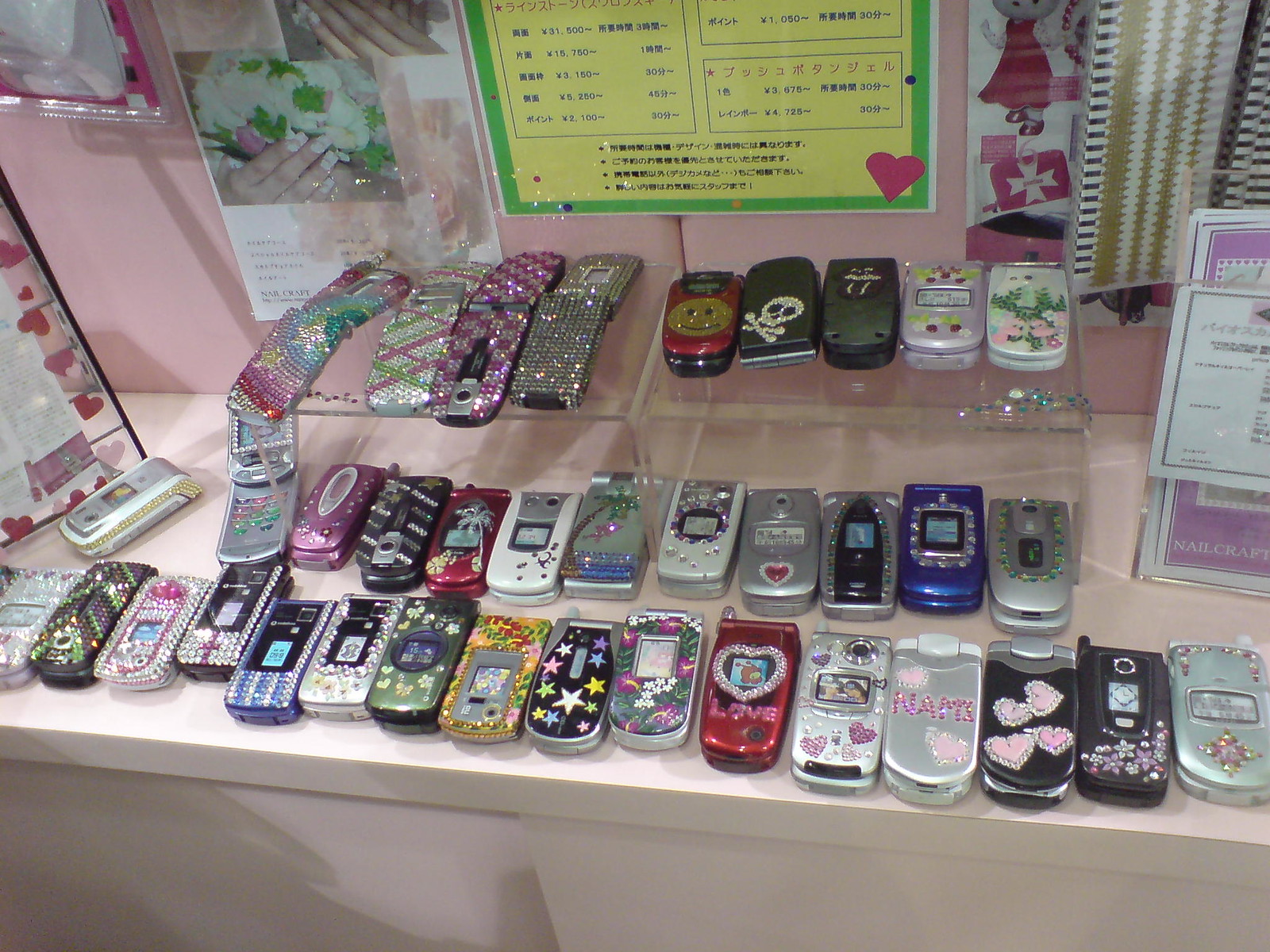The image displays over 30 uniquely customized flip phones arranged on a brightly colored counter, either yellow or pink. The backdrop features a vivid pink wall adorned with various pictures, posters, and notes. On both the left and right sides of the display, there are acrylic stand-up displays with paperwork. The flip phones themselves are situated in two rows on the counter, with additional rows on each of the two acrylic holders flanking either side.

Each acrylic holder contains a row of flip phones, all open to showcase their adorned cases. On the left holder, four flip phones gleam with sparkly rhinestone cases. The right holder displays five flip phones, including a distinctive red one with a yellow smiley face, several black ones, a lavender phone displaying its screen, and a white one. The cases of these phones are embellished with an array of decorations, including rhinestones, hearts, stars, and stickers, and come in a variety of colors such as blues, yellows, greens, silvers, reds, blacks, and notably, pink. The customization and personalization of each phone highlight their unique designs and suggest that they were once beloved personal items. The overall display gives the impression of being a vibrant showcase, possibly for sale or exhibition.